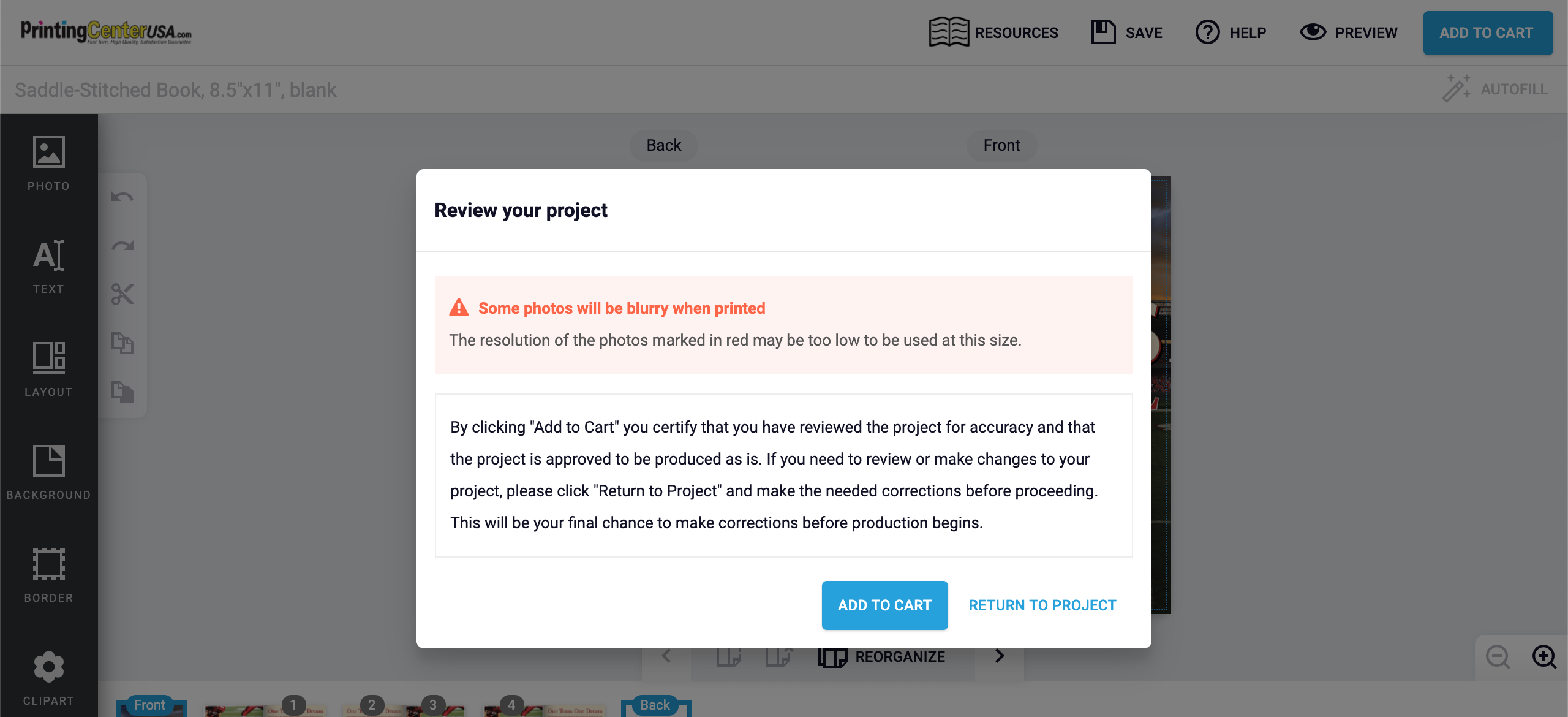This screenshot features a notification on the printingcenterusa.com website. In the top left corner, the company name "PrintingCenterUSA.com" is prominently displayed. Adjacent to this, in the top right-hand corner, there are several buttons and icons: a blue "Add to Cart" button with white letters, a "Resources" tab represented by a book icon, a "Save" option illustrated by a floppy disk icon, a "Help" function marked by a question mark within a circle, and a "Preview" option featuring an eye icon.

At the center of the screenshot, a detailed notification is shown within a white box. The box's header, in black lettering, reads "Review Your Project." Directly below, a light pink rectangle alerts users with an orange triangle icon and text that states, "Some photos will be blurry when printed." Further, it warns, "The resolution of the photos marked in red may be too low to be used at this size."

The notification continues with a paragraph informing users that by clicking the "Add to Cart" button, they certify they have reviewed the project for accuracy and approve its production. It advises that if any revisions are necessary, they should click "Return to Project" to make corrections before proceeding, highlighting this as the final opportunity for changes before production begins.

Beneath this text, there are two additional buttons: a blue "Add to Cart" button and a white "Return to Project" button with blue lettering.